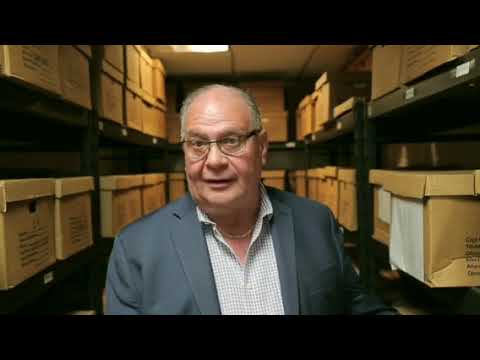In the image, an older, Caucasian man is seen standing inside a storage closet or file room, framed by thick black borders at the top and bottom. The storage area contains black metal shelves filled with brown banker’s boxes, which are stacked two layers high on the left side. The boxes have lift-off lids and handles for carrying. The man, positioned from the upper chest upwards at the center of the image, appears to be looking directly at the camera with his mouth slightly open as if speaking. He is balding, with short gray hair on the sides, and wears thin-rimmed glasses. His face is round with rosy cheeks and thick jowls. He dons a light gray dress jacket over a collared, light blue, gray, and white checkered shirt, with a thin gold necklace around his neck. The room is lit by a single fluorescent light, enhancing the detailed textures and colors in the close confines of the storage space.